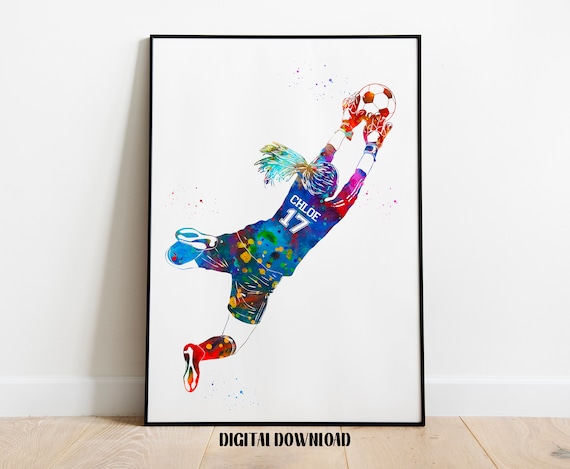In this vibrant and colorful painting, a female soccer goalie is captured mid-action, reaching up to block a red and white soccer ball. The artwork is framed with a thin black frame and positioned against a pristine white wall, casting a dark gray shadow. The floor beneath is made of beige wood panels, and beneath the frame, bold black text reads "digital download."

The goalie is depicted with her hair pulled back in a ponytail that is vibrantly mixed with turquoise, yellow, and purple hues. Her face is magenta, and she wears a predominantly blue jersey with red arms and pink sleeves. The back of her jersey prominently displays the name "Chloe" and the number "17." Her shorts are a teal color adorned with green, purple, and yellow splotches, and she sports knee-high socks in a variety of colors, along with soccer cleats. The overall composition of the painting is a stunning collage of multicolored splashes and patterns, adding a dynamic and energetic feel to the scene.